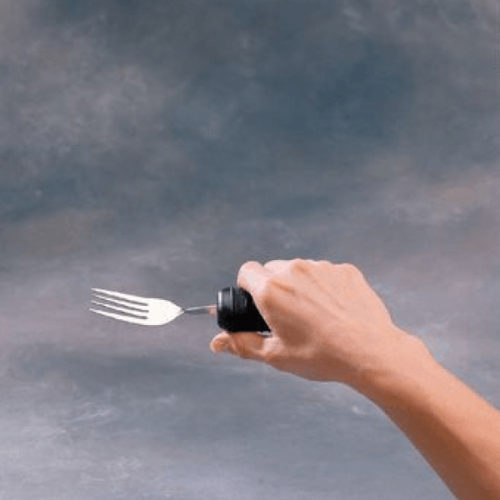The image depicts a person's right hand and forearm emerging from the lower right corner and extending towards the center. The hand holds a silver fork with four prongs, but what stands out is that the fork is attached to a round, cylindrical black object gripped in the person's hand. The thumb is positioned on the underside while the other fingers curl over the top. The background is a blend of light gray, dark gray, and white, resembling a misty, cloudy sky, giving it a consistent and soft appearance throughout. The black object holding the fork could be a stabilization device, possibly used by individuals with shaky hands to aid in eating independently. The image has no text.